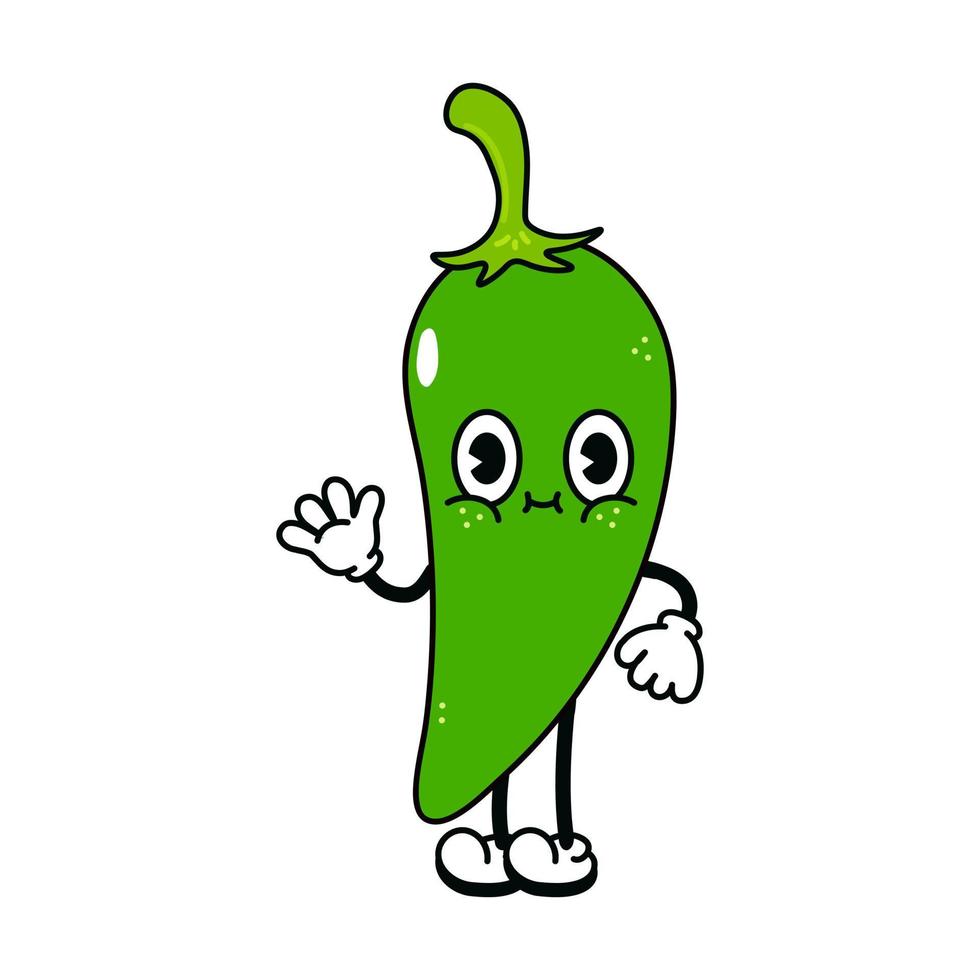This digital cartoon illustration features "Mr. Jalapeno," a lively and anthropomorphized green jalapeno pepper. Mr. Jalapeno is depicted with a recognizable curved shape, leaning slightly to the left, and topped with a lighter green stem. His expressive face includes big, bright eyes with Pac-Man-shaped black pupils surrounded by white, and puffy cheeks indicated by little lines underneath. A slight smile is visible between the eyes. He also has three yellow dots under his cheeks, resembling dimples. The character’s arms are extended, with the right arm waving hello and the left arm resting downward, each ending in a white cartoon glove with a thumb and three fingers. Mr. Jalapeno is further animated with two thin black legs that resemble toothpicks, each sporting cartoonish shoes. Set against a plain white background with no caption or frame, this illustration portrays a welcoming, cheerful green pepper waving to the viewer.